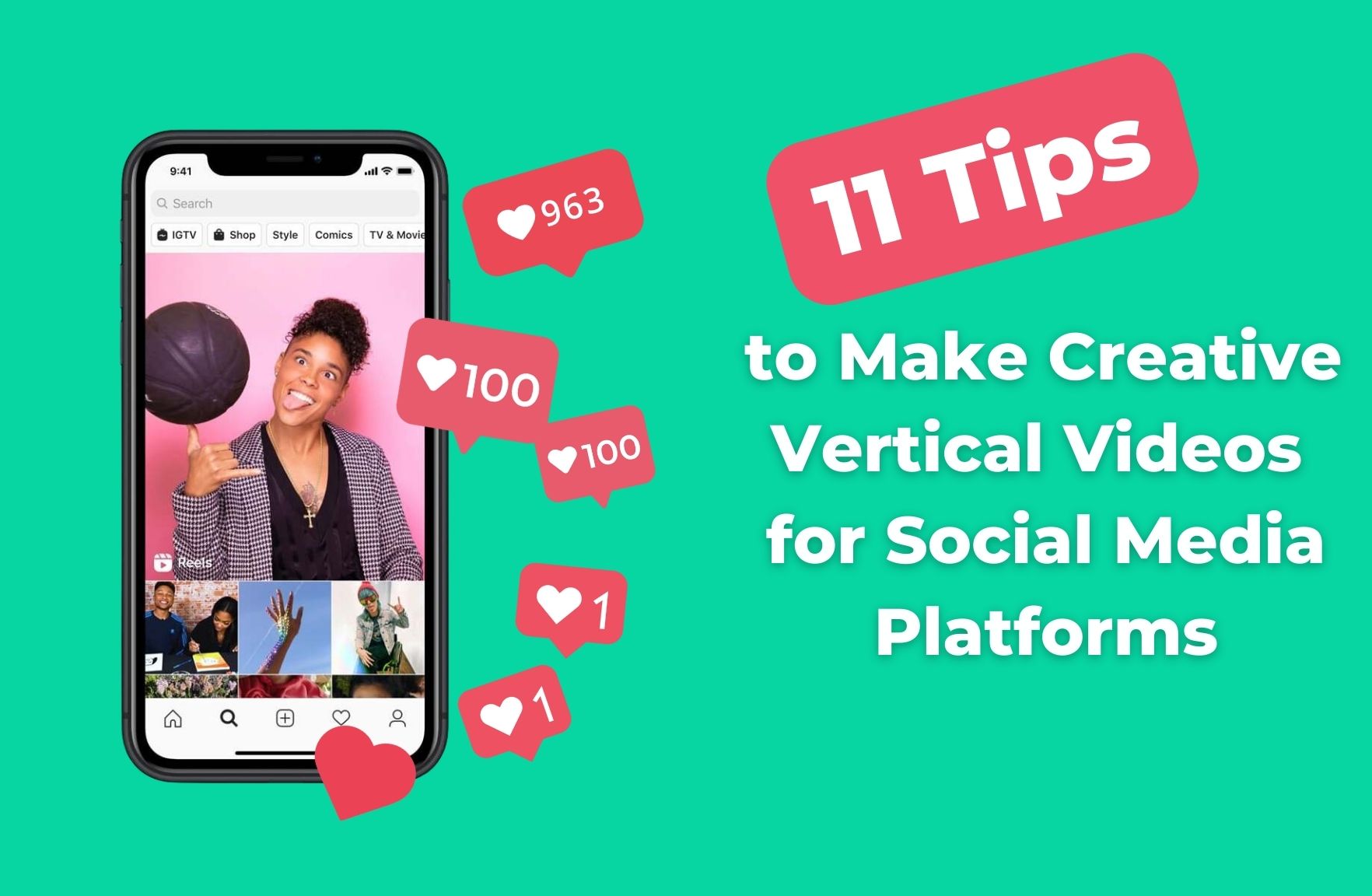This image, likely a thumbnail for a YouTube video advertisement, is designed to promote an instructional guide titled "11 Tips to Make Creative Vertical Videos for Social Media Platforms." The layout features a light green background with a phone display on the left side. The phone screen shows a dark-skinned woman with a tattoo on her chest, a cross necklace, a black checkered jacket, and a black v-neck shirt, skillfully balancing a basketball on her thumb while sticking out her tongue. Above her image, red bubbles indicate social media likes: one shows "963" with a heart, another "100" with a heart, a smaller "1" with a heart, and another "1" with a heart, emphasizing the engagement potential of vertical videos. To the right, bold red text at the center of the image reads "11 Tips" with white lettering beneath it stating "to make creative vertical videos for social media platforms." Additional minor images on the phone screen include a gesture of hands with a rainbow pattern and two African-American individuals, a man and a woman, examining a book together, further showcasing dynamic and engaging content.